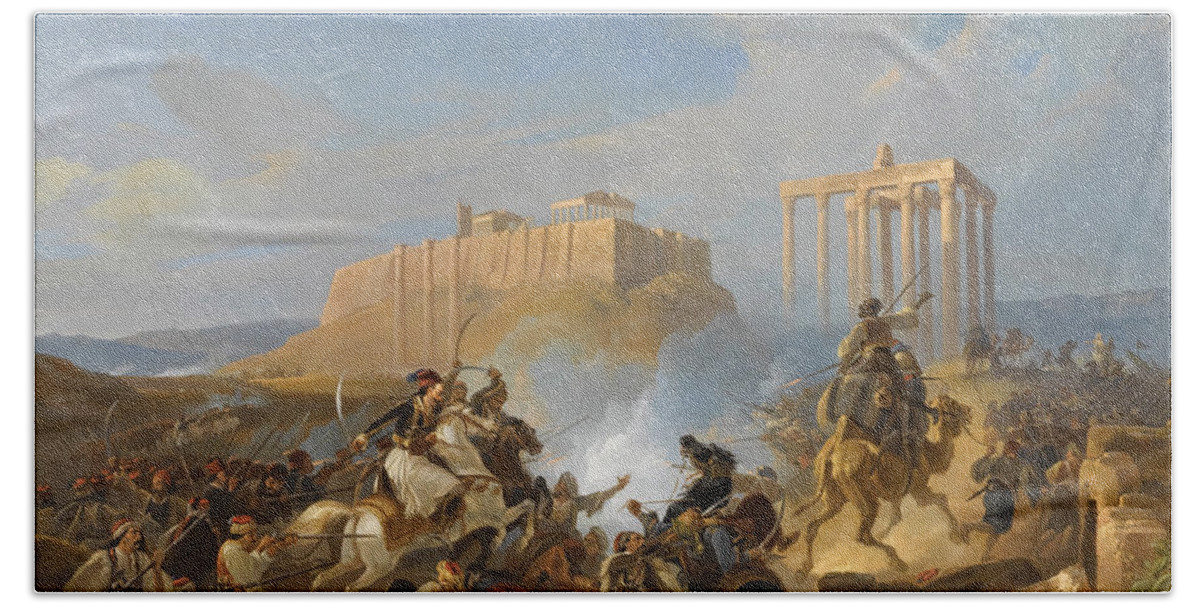This detailed horizontal painting, possibly a reprint on a blanket with stitched borders, portrays an intense battle in a desert-like setting, likely in ancient Greek or Mediterranean times. The bottom half is a chaotic melee of warriors wielding swords, spears, and rifles. On the right, there's a black man riding a camel, appearing either to retreat or flee from the battle, along with others retreating over the sandy terrain. In contrast, soldiers on the left, mounted on white horses, are charging forward, brandishing their swords aggressively. A dense column of white smoke rises from the center of the battlefield, adding to the scene's intensity. The backdrop features a massive rocky plateau, crowned with a fortified stone structure resembling ancient Athens architecture. To the right of this plateau stands a robust stone columned structure. Above all of this, the sky is painted a light blue, adorned with thin white clouds, encapsulating the historic and tumultuous atmosphere.